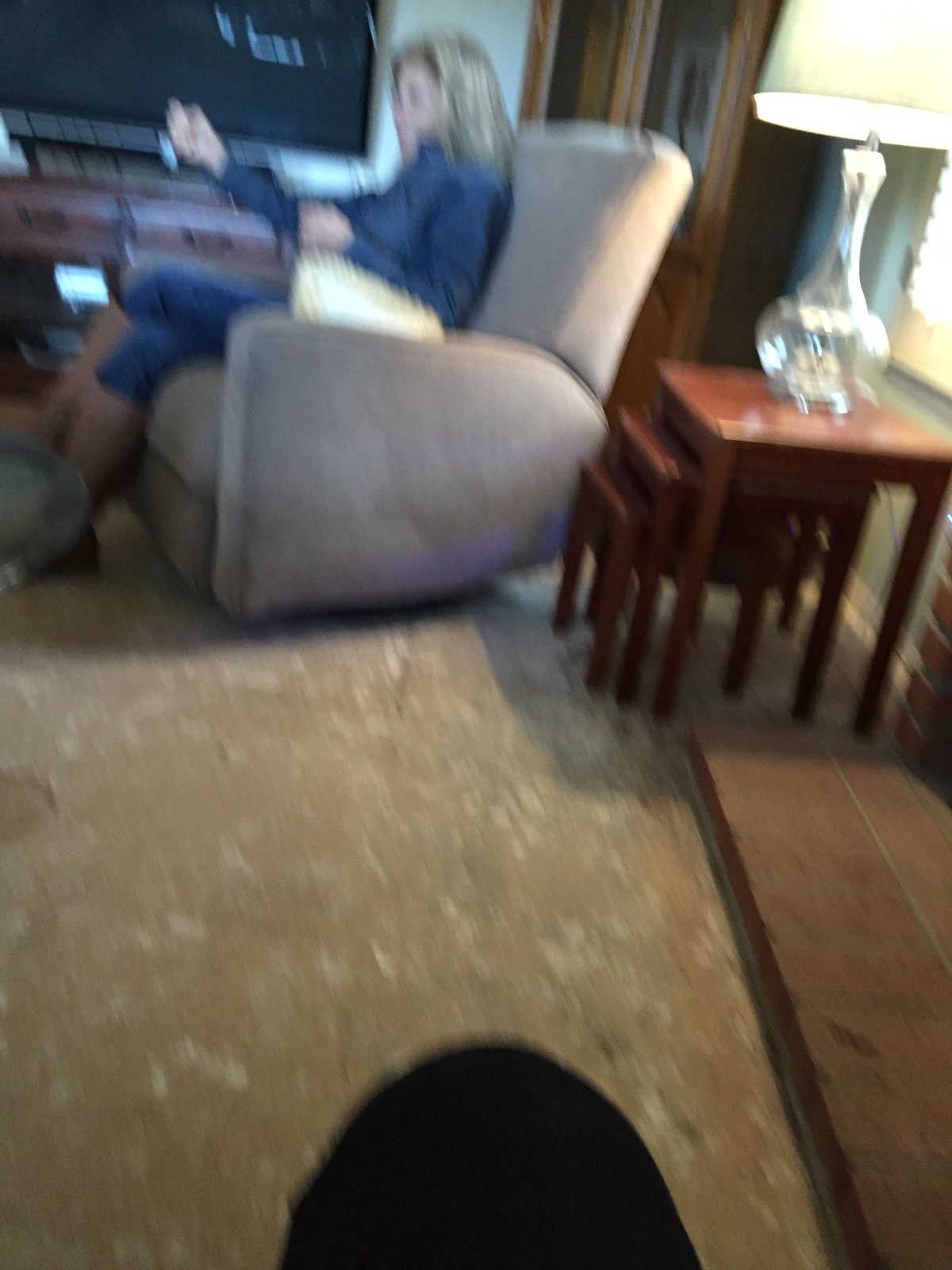In this image, a cozy living room is depicted with a lady as the central focus. She is seated comfortably in a large light beige reclining chair. The woman is blonde with long hair and is dressed in a blue jean outfit paired with beige-colored boots, exuding a casual yet stylish look. To her right stands a large green television on a stand, contributing to the room's entertainment setup.

Behind her, a substantial shelving unit with two glass doors is visible, hinting at storage or display space. In front of a window, there are nesting tables arranged neatly - a set of three tables that fit into each other. These tables support a lamp with a clear base and a white shade, adding a touch of elegance to the scene.

The flooring of the room features a mix of textures; in the background, there are visible sections of brick, while the foreground showcases brown and white tiled flooring. The shadow of a table falls across the tiles, adding depth and dimension to the image.